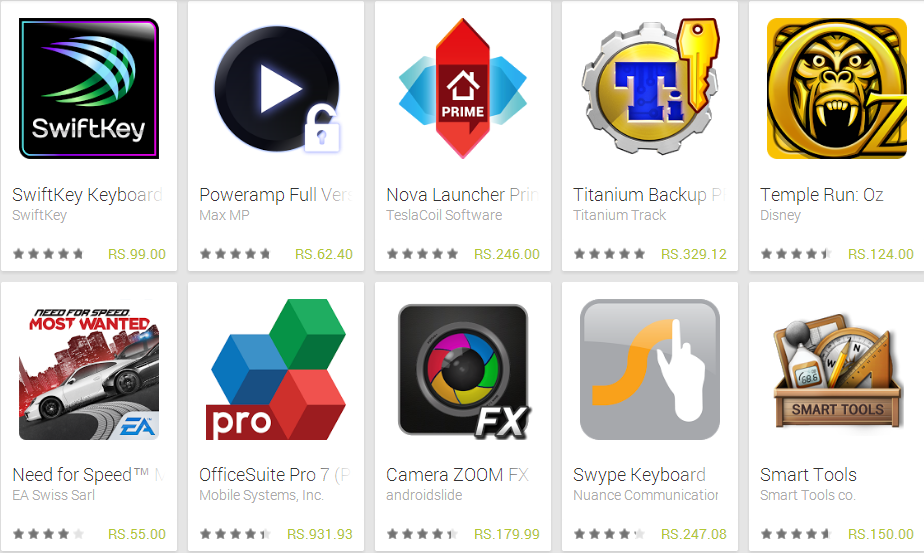This image showcases a collection of popular website logos, each accompanied by star ratings, organized in two rows.

In the upper left corner, the first logo is for SwiftKey, displayed on a black square with a green swirling design. The caption reads "SwiftKey Keyboard, 5 stars." Following this is a logo within a black circle featuring a white arrow pointing to the right. Next, within another black circle, is a white unlocked padlock, labeled "PowerRamp, 5 stars."

Continuing, there is a logo that reads "Prime" decorated with a pink arrow pointing up and down, and within a square center, a white house frame with blue designs on each side. The text below reads "Nova Launcher." This is followed by a circle containing the letters "TI" and a key, representing "Titanium Backup."

Next, a logo with "Oz" and the face of an ape in the center is accompanied by the caption "Temple Run, Oz Disney, 4.5 stars." 

Moving to the lower row, the first logo is for "Need for Speed, Most Wanted," featuring a depiction of a white car below it. The text includes "Need for Speed, EA, Swiss, S-A-R-I, 4 stars." 

Following this is a logo labeled "Pro," composed of block designs in blue, green, and red, with the text "Office Suite Pro 7, Mobile Systems Inc., 4.5 stars" below. 

Another logo reads "FX" and includes a camera lens with colorful edges in red, pink, blue, green, and yellow. It is described as "Camera Zoom FX, Android Slide, 4.5 stars."

Next is a gray button with a white hand making a blue swirling mark, the thumb and index finger pointing upward. The caption reads "Swipe Keyboard, Nuance Communication, 4 stars." 

Lastly, the "Smart Tools" logo features a small box filled with tools, including a compass and a pencil, and is labeled "Smart Tools Company."